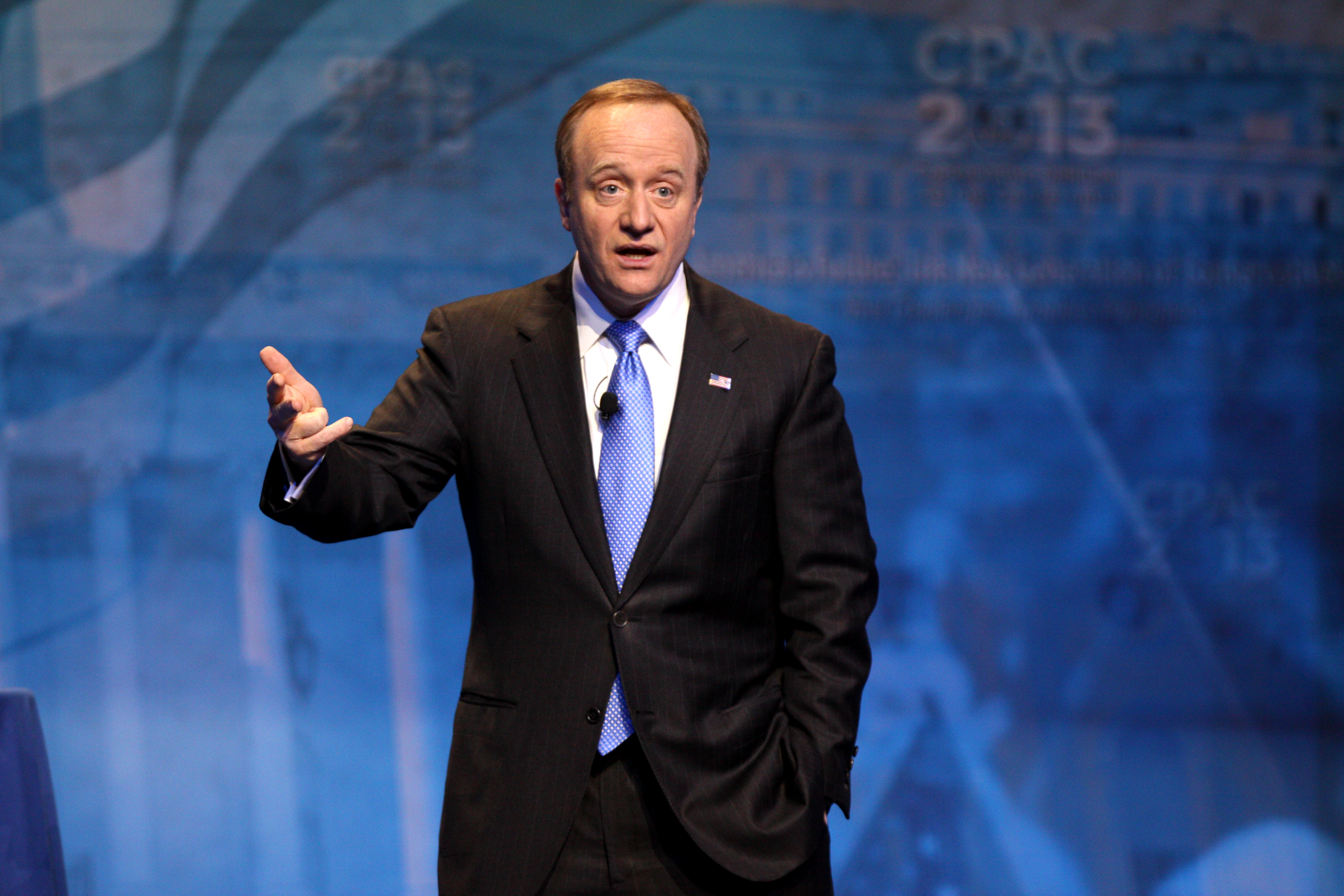The photograph captures a middle-aged white male, likely in his late 40s or 50s, who is clean-shaven with short, brown hair neatly combed to the side. He is wearing a black suit with a white undershirt and a blue tie adorned with white dots. An American flag pin is fastened to his left lapel, and a microphone is clipped to his tie. The man is positioned centrally in the image, seen from the hips upwards with his left hand in his pant pocket and his right hand raised, appearing to address a crowd. His eyes are wide open, eyebrows raised, and his mouth is open, mid-speech.

He stands against a vibrant blue background, filled with various light blue, white, and gray graphics. Prominently displayed is the text "CPAC 2013," indicating the event, along with elements resembling an American flag and possibly images of buildings. The setting suggests an indoor conference held during the day.